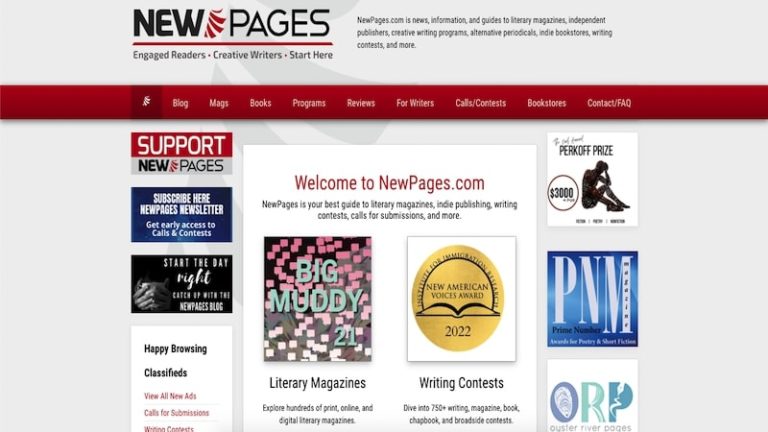Sure, here's a cleaned-up and detailed caption for the image:

---

The "New Pages" section of a newspaper or news website features a prominently displayed header with the title "New Pages" at the top. Directly below, a bold red navigation bar lists various menu options including "Blog," "Mags," "Books," "Programs," "Reviews," "For Providers," "Calls," "Book Stories," and "Contact/Frequently Asked Questions." Beneath this bar, readers are greeted with a welcoming message from NewPages.com, accompanied by a link to a blogging contest, inviting participation. To the left of this welcome message, there is a clickable link titled "Big Muddy 21," potentially leading to a highlighted article or feature. To the right, three additional clickable tiles are displayed, though their specific content or destinations are unclear.

---

This description should provide a clear and detailed understanding of the image.